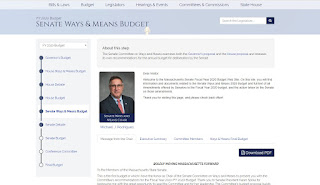The image depicts a web interface with a prominent white search bar at the top center of the screen. To the left of the search bar, there is an area featuring various lines of text, although the specific content is partly obscured and difficult to read. There seems to be a label or link that includes the phrase "About this," suggesting information or navigation options related to the page or topic.

In the middle of the screen, there is a figure illustrated with a high level of detail. This person is wearing a black suit paired with a red tie and glasses, giving them a professional appearance. The right side of the image is notably pixelated, making it challenging to discern specific details clearly. However, it appears to include a button or link labeled "Download PDF," along with additional text elements that are similarly distorted and unreadable.

Overall, the image gives an impression of a website with a somewhat cluttered and pixelated design, making precise comprehension difficult. The person in the center stands out as the most readily identifiable element, set against a background of various textual and navigational components.